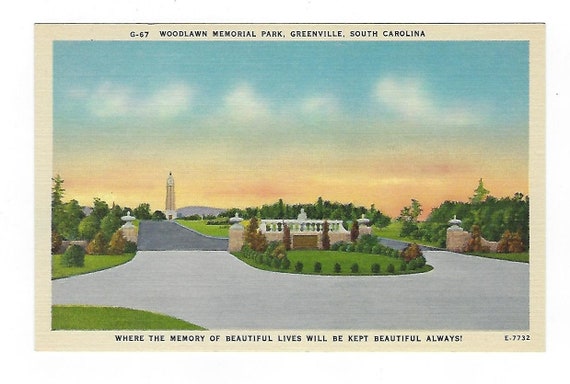This detailed concept drawing of the Woodlawn Memorial Park in Greenville, South Carolina, features a tan-colored frame with inscriptions. At the top, the frame reads "G67 Woodlawn Memorial Park, Greenville, South Carolina," while the bottom bears the poignant phrase "where the memory of beautiful lives will be kept beautiful always," along with the identifier "E772" on the lower right. The scene within shows a landscaped memorial area with a mixture of concrete pathways branching out to the left, back, and right. Central to the image is an oval expanse of green grass bordered by bushes and a low white railing, with a figure standing nearby. This area leads to a rounded building with predominantly tan and white colors. On the side, a small tower resembling part of a gate adds a touch of architectural interest. Surrounding the memorial are trees and a background characterized by a gently rolling hill. The sky above transitions from a warm mix of orange and yellow hues at the horizon, suggesting either dawn or dusk, to a serene blue higher up, dotted with a few clouds. The entire image has a hand-drawn quality, enhanced with color, giving it the appearance of a thoughtfully designed postcard or concept artwork.